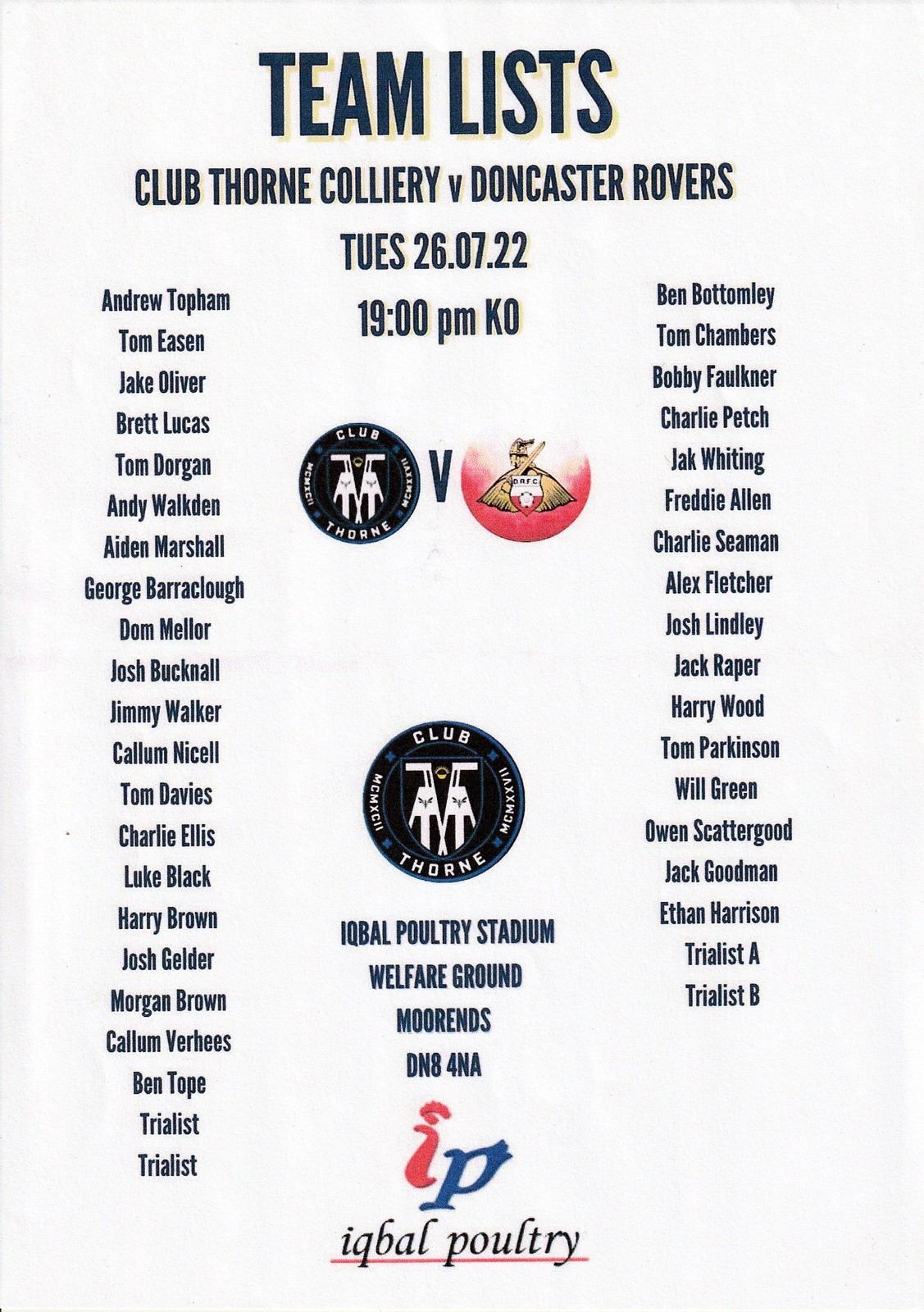This image is a vertical poster titled "Team Lists," presenting a detailed layout of two British football teams: Clubthorn Colliery and Doncaster Rovers. The background is white, and all text is in black. Beneath the title, the event details are listed: "Clubthorn Colliery v. Doncaster Rovers, Tuesday 26.07.22," with the match scheduled for "19:00 p.m. KO." The poster features two columns of player names, with the left column listing 22 names for Clubthorn Colliery, and the right column listing 18 names for Doncaster Rovers.

Between the columns, the clubs' symbols are displayed prominently. Clubthorn's symbol, which resembles two blocky figures with hockey sticks, appears above and below the list, with the text "Club Thorn" accompanying it. The Doncaster Rovers' symbol, resembling a tiki hut with a shield, is also featured.

At the bottom of the poster, additional details about the venue are provided: "Iqbal Poultry Stadium, Welfare Ground, Moran's, DN8-4NA." The Iqbal Poultry logo appears beneath this text, completing the design of the poster.